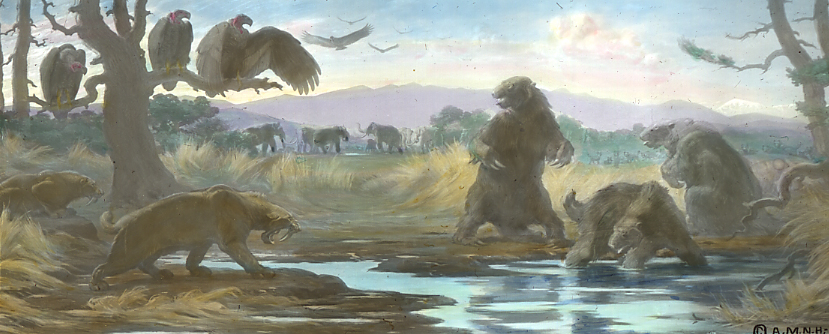This detailed watercolor painting illustrates a dramatic prehistoric scene at a watering hole. In the foreground on the left, two saber-toothed tigers are baring their teeth at three bear-like creatures with long claws and abundant fur on the right. One of these creatures is poised on its hind legs, while the other two stand on all fours, one even positioned in the water. 

Dominating the upper left, a large tree hosts several ominous vulture-like birds, hunched over and staring intently at the unfolding standoff. More of these birds are seen circling in the bright blue sky filled with puffy white clouds above. Spanning the background, a majestic mountain range rises, adding depth to the image, with a herd of mastodons visible in the distance, reinforcing the prehistoric setting. 

Nestled in the bottom right corner is the artist's signature, though it's not entirely legible, marking this as a signed work of art. This illustration blends dynamic animal interactions with rich environmental details, capturing the ancient ecosystem in vivid detail.